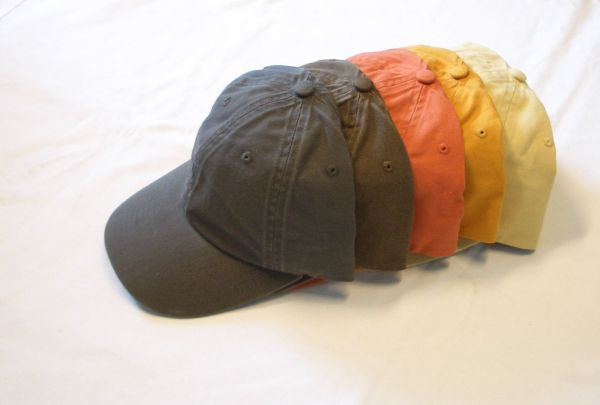The photograph features five ball caps meticulously arranged on a creamy white background, possibly a bedsheet or similar fabric. The caps are stacked from the lower left to the upper right, folded in half so that the back half of each cap is tucked into the front, significantly reducing the size of the head covering area. They are positioned with their brims facing the lower left corner and the flattened backs towards the upper right.

Starting from the lower left, the sequence of caps includes:
1. A charcoal gray cap
2. Another charcoal gray cap
3. A tangerine orange (or bright coral) cap
4. A mustardy yellow (or off yellow) cap
5. A creamy white cap with a hint of light yellow

Each cap features the characteristic button on the center of the dome, and although they vary in color, their structure is identical. The arrangement creates a gradient effect, progressing from darker to lighter shades, and emphasizes the visual harmony of the neatly stacked and uniformly folded caps.